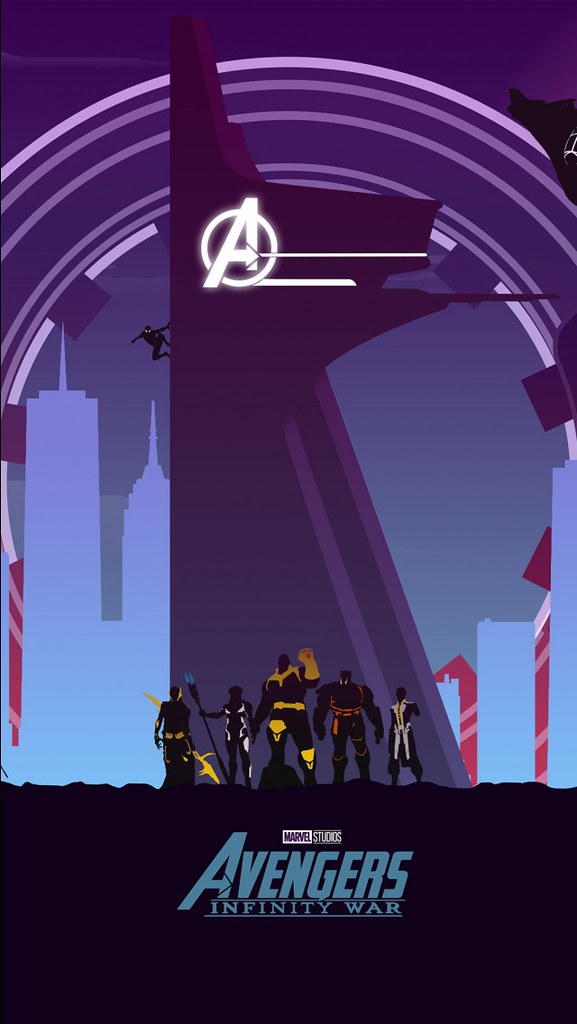This detailed poster for Marvel Studios' "Avengers: Infinity War" is computer-animated and features vibrant hues of blue, purple, and red. Dominating the background is a tall building, purportedly the Avengers complex, marked by a prominent white 'A' with a circle around it near the top. This building extends outward on the right side, possibly forming a landing pad. In front of this structure stand several characters, dressed distinctively, presumably the Avengers. One character in black attire is distinguished by gold gloves and knee pads, while another character to the left wields a long stick. A smaller, black figure is visible at the top of the building, suggesting a climactic moment. The bottom of the poster features the title "Avengers: Infinity War" in blue letters, with "Marvel Studios" inscribed above it, emphasizing the epic and heroic nature of the scene. The overall style is cartoony yet impactful, capturing the grandeur of the movie's theme.